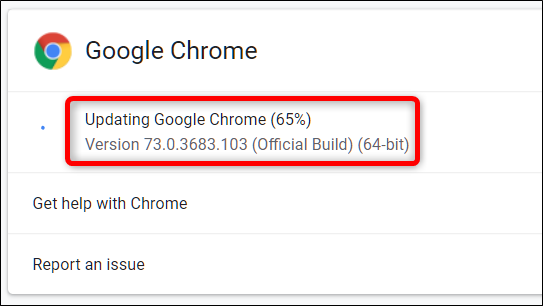The image is a screenshot of a website, featuring a rectangular element with a thin black border outlining the perimeter. Inside the rectangle, there is a gray-colored top, left side, and bottom margin, while the central area showcases a white background. Positioned at the top left of this background is an icon that consists of a circle divided into sections with different colors – blue in the center, red at the top, green on the left, and yellow on the right, representing the Google Chrome logo. 

To the right of the icon, the text "Google Chrome" is displayed, with the letters 'G' and 'C' capitalized and the text appearing in a larger, bold font. 

Below this header, a horizontal line is followed by a blue circular icon, after which the text "Updating Google Chrome" appears with "65%" in parentheses adjacent to it. 

Underneath this, the version information is provided as "Version 73.0.3683.103", with "Official Build" in parentheses where the 'O' and 'B' are capitalized. Additional information "(64-bit)" is also provided next to it. This block of text is outlined by a red line. 

Further down, another horizontal line precedes the text "Get Help With Chrome," with both 'G' and 'C' capitalized. Finally, another line is followed by the text "Report an Issue," where 'R' is capitalized.